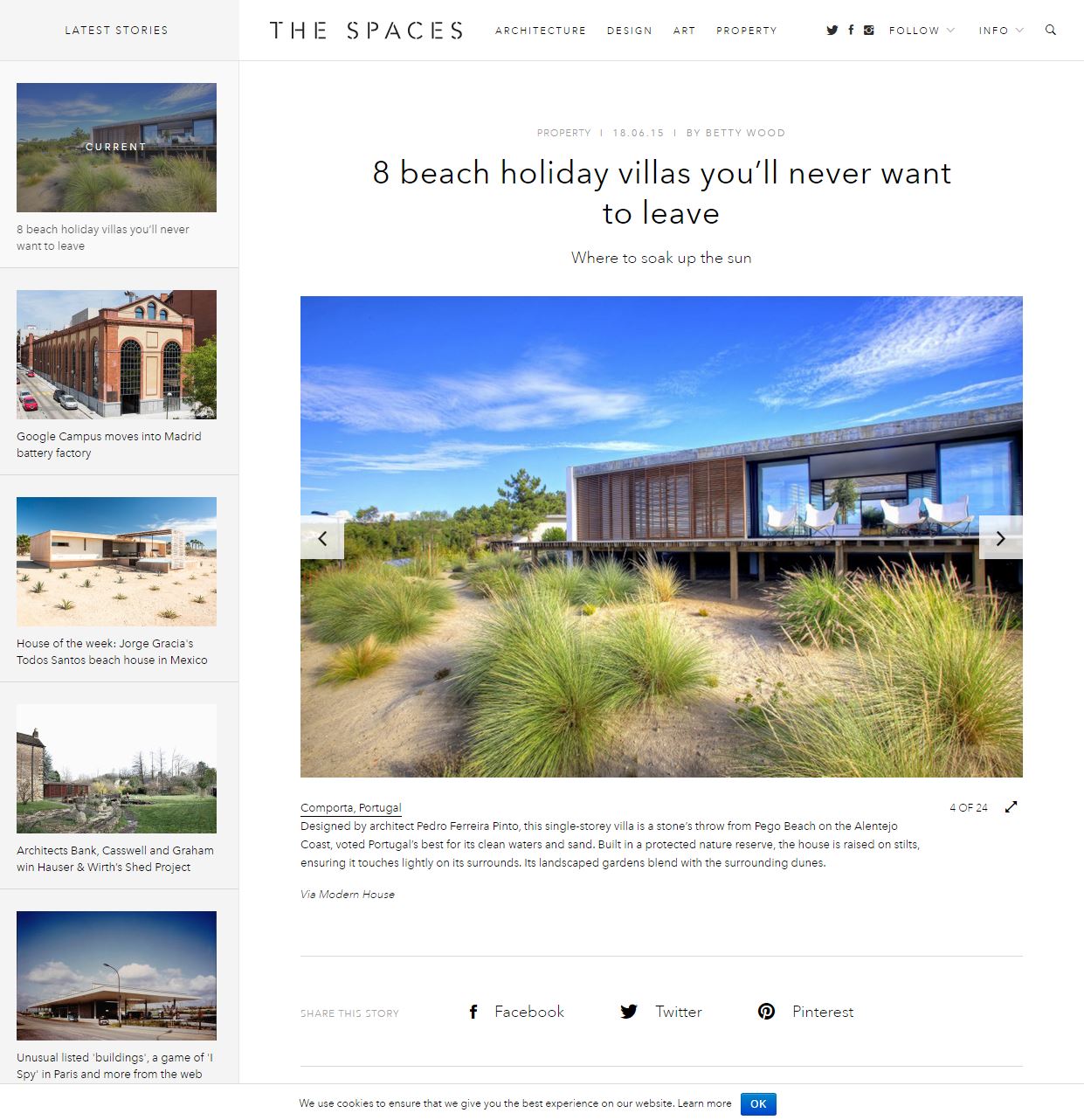This is a detailed screenshot capture of a real estate webpage with a predominantly white background. On the left-hand side, there's a sidebar titled "Latest Stories," showcasing five square image blocks each corresponding to various stories. 

1. The first block features an inviting beach scene with the headline: "8 Beach Holiday Villas You'll Never Want to Leave." A picturesque beach is depicted underneath the title.
2. The second block presents an urban setting with brick buildings and cars lining the streets. The headline reads: "Google Campus Moves into Madrid Battery Factory."
3. The third block shows what seems to be a trailer by the beach, accompanied by the title: "House of the Week - Hey Gracias Todos Santos Beach House in Mexico."
4. The fourth block depicts a green field with some bare trees and a brick wall, titled: "Architects Bank Caswell Graham with Hauser and Workshed Project."
5. The fifth and final block illustrates a business building with an extended awning, set against a blue sky. The headline is: "Unusual Listed Buildings: A Game of I Spy in Paris and More from the Web."

Central to the webpage is the title in bold black letters, "8 Beach Holiday Villas You'll Never Want to Leave," with a subheading inviting readers to "soak up the sun." Below this title is a striking image of a unique beach house elevated on stilts. The house is nestled on a sandy beach bordered by lush, spiky green plants and backed by a grove of trees. The location is noted underneath as Comporta, Portugal.